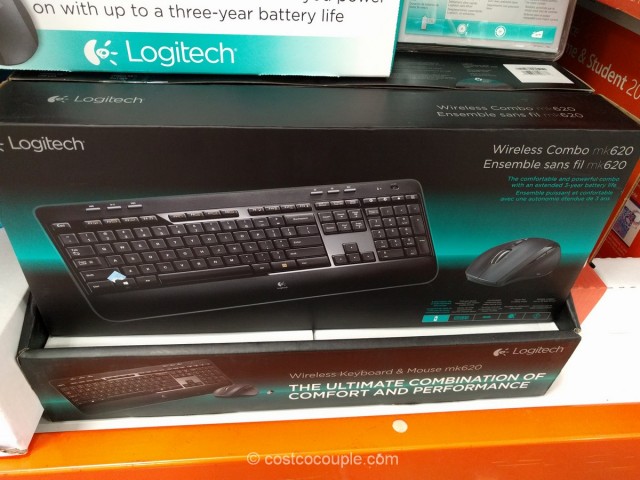In this image taken inside a department or electronics store, there is a prominently displayed section featuring an array of wireless keyboard and mouse combos from the popular brand Logitech. The top part of the image showcases the lower half of a green and white box labeled "Logitech." In the central portion of the image, as well as towards the bottom, there are several black and green boxes depicting a black keyboard and wireless mouse combo. Each box is branded with "Wireless Combo MK620" in the upper right corner, followed by a Spanish translation underneath. The front of the boxes vividly displays images of the keyboard and mouse. Additionally, in the top right corner of the image, there's a red box with white text related to students and a number. On one of the Logitech boxes, a marketing tagline reads, "The ultimate combination of comfort and performance," emphasizing the product's quality and ergonomic design.